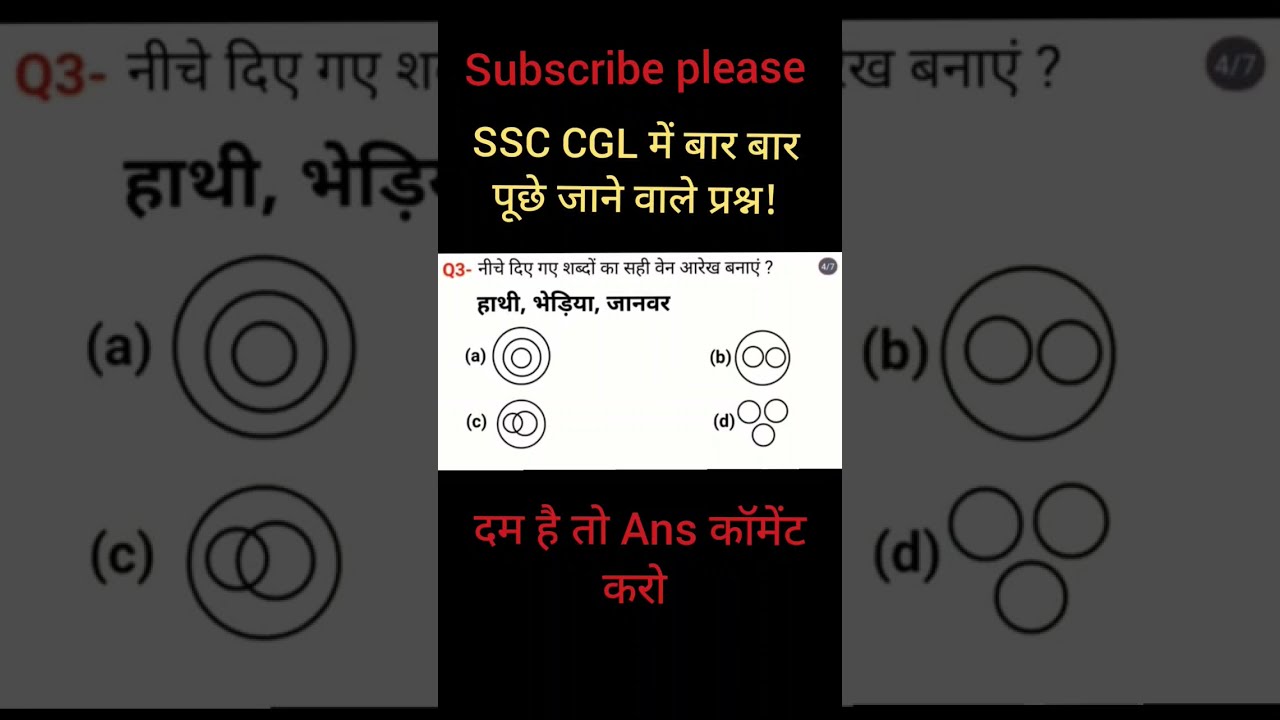The image is a long, vertical landscape featuring a prominent equation written in a different language, bracketed by two large black sections. The upper black section in the center includes English text stating "subscribe please" in red, followed by "SSCCGL" in yellow, accompanied by unrecognized Middle Eastern characters ending in an exclamation point. The lower black section also contains Middle Eastern script. Surrounding the central equation are semi-transparent, zoomed-in copies of the image, grayish in tone, filling the negative space to the left and right. In the lower part of the central section, amid more Middle Eastern characters, the characters "AMS" and "Q3" appear, with four potential answer options. There is also some text in Arabic and distinctive circular shapes. The overall image appears as a math problem or educational graphic.